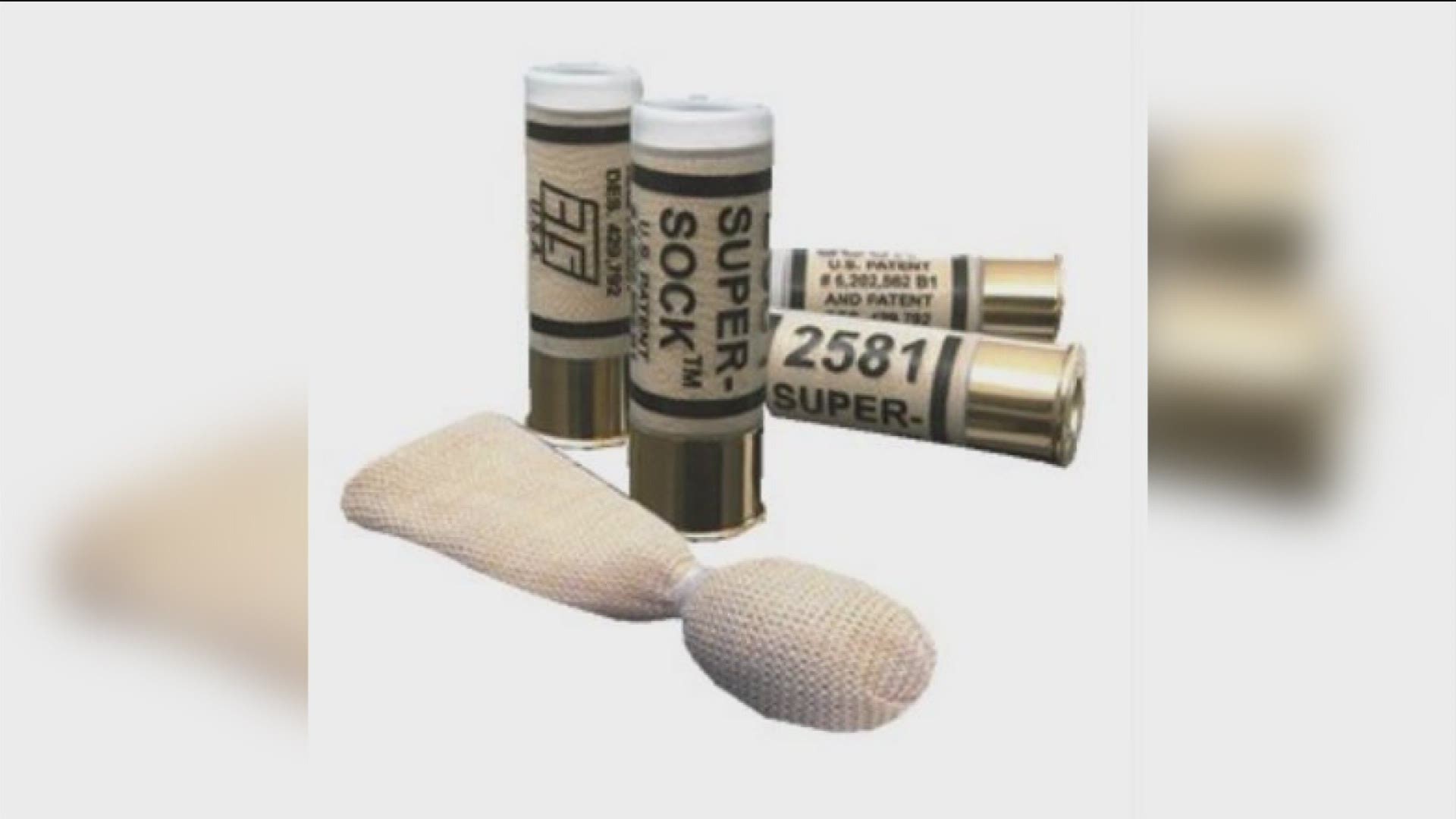The image depicts four small, capsule-like objects with a gold base and white top, each labeled with the text "Super Sock" and the code "2581." The capsules, resembling bullet casings, are positioned against a white backdrop with blurred edges creating a photographic effect. Two of the capsules are standing upright while the other two lie horizontally. In the foreground, there is a beige fabric or sock emerging from one of the capsules, featuring a circular top and a triangular bottom, giving it a somewhat humanoid appearance. This fabric is tied in a ball at one end. A black and beige label on the capsules is partially visible, and a U.S. patent number is mentioned.